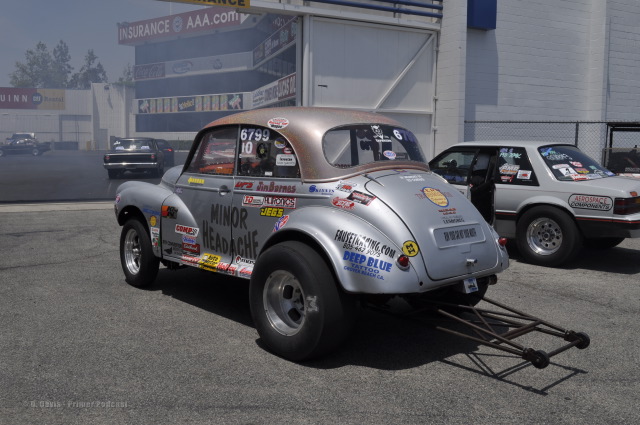In the image, a collection of vintage cars are seen lined up on the road. Dominating the scene at the center is a uniquely decorated vintage car in shades of gray and silver-green. This car is adorned with an array of text and logos scattered across various parts of its body, including doors, bonnets, and windows. Prominent inscriptions include "Minor Headache," "Jax," and "679910," along with numerous colorful logos. Near the rear light area, logos such as "FaucetCarrying.com," "8054679073," and "DeepBlueTattoo" are visible. The car’s vehicle number remains unclear, and an additional trolley appears to be attached below it.

On the right side of the image, another gray vintage car comes into view, similarly embellished with logos and stickers. In the background, a massive building towers over the scene, displaying banners at multiple levels. The top level features a legible banner reading "InsuranceAAA.com," while the other banners are not clearly discernible. Additional vintage cars are parked in front of this building. The atmosphere appears somewhat hazy, with a wall in the background showing a barely readable hoarding with the letters "UINN." Beyond this, trees are faintly visible.

Daylight illuminates the scene, casting shadows of the cars onto the road, and creating a clear, vibrant ambiance. The bottom-left corner of the image contains a faint footnote that is not easily readable.